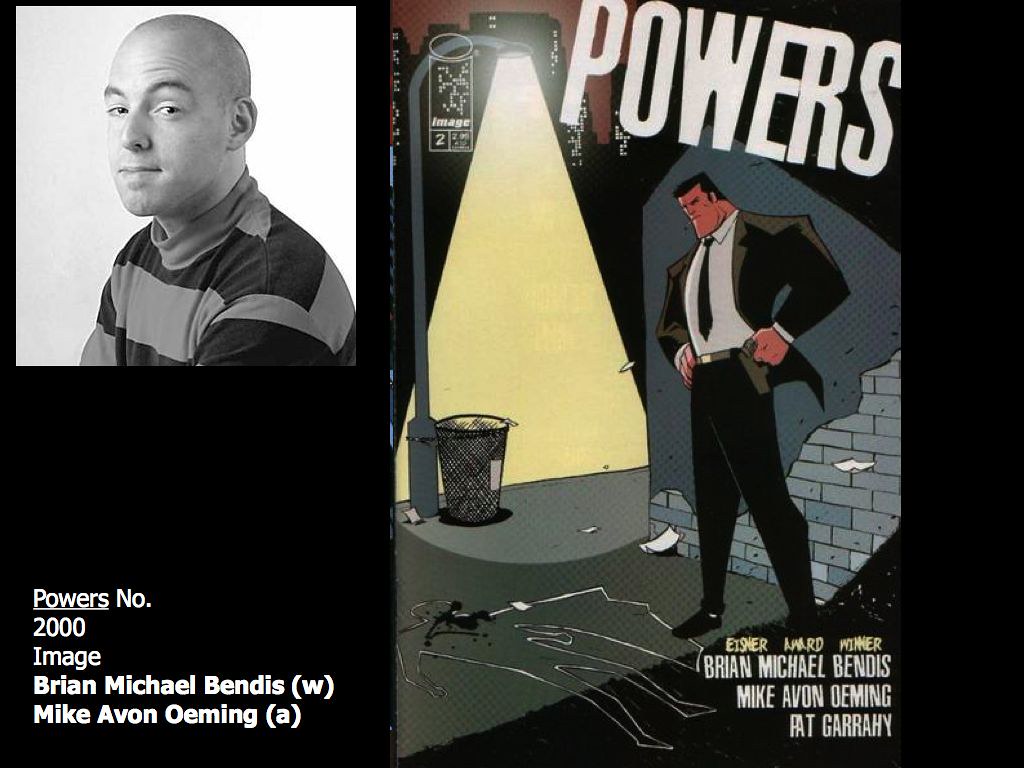This is an image of the cover of the comic book "Powers," issue number 2, published by Image Comics in 2000. On the left side of the cover, there is a black and white photograph of a man in a dark and white striped shirt, who is presumably either Brian Michael Bendis, the writer (denoted by the W), or Mike Avon Oeming, the artist (denoted by the A). The man is bald and looking at the camera with a neutral expression. 

On the right side, the front cover features a detailed graphic drawing that focuses on a detective or police officer dressed in a suit and tie. His hand rests on his pistol as he intently examines a chalk outline on the ground where a dead body apparently was. The scene is illuminated by a street lamp, casting light on the surrounding area, which includes some blood stains and a nearby garbage can. The title "Powers" is prominently displayed at the top of the cover.